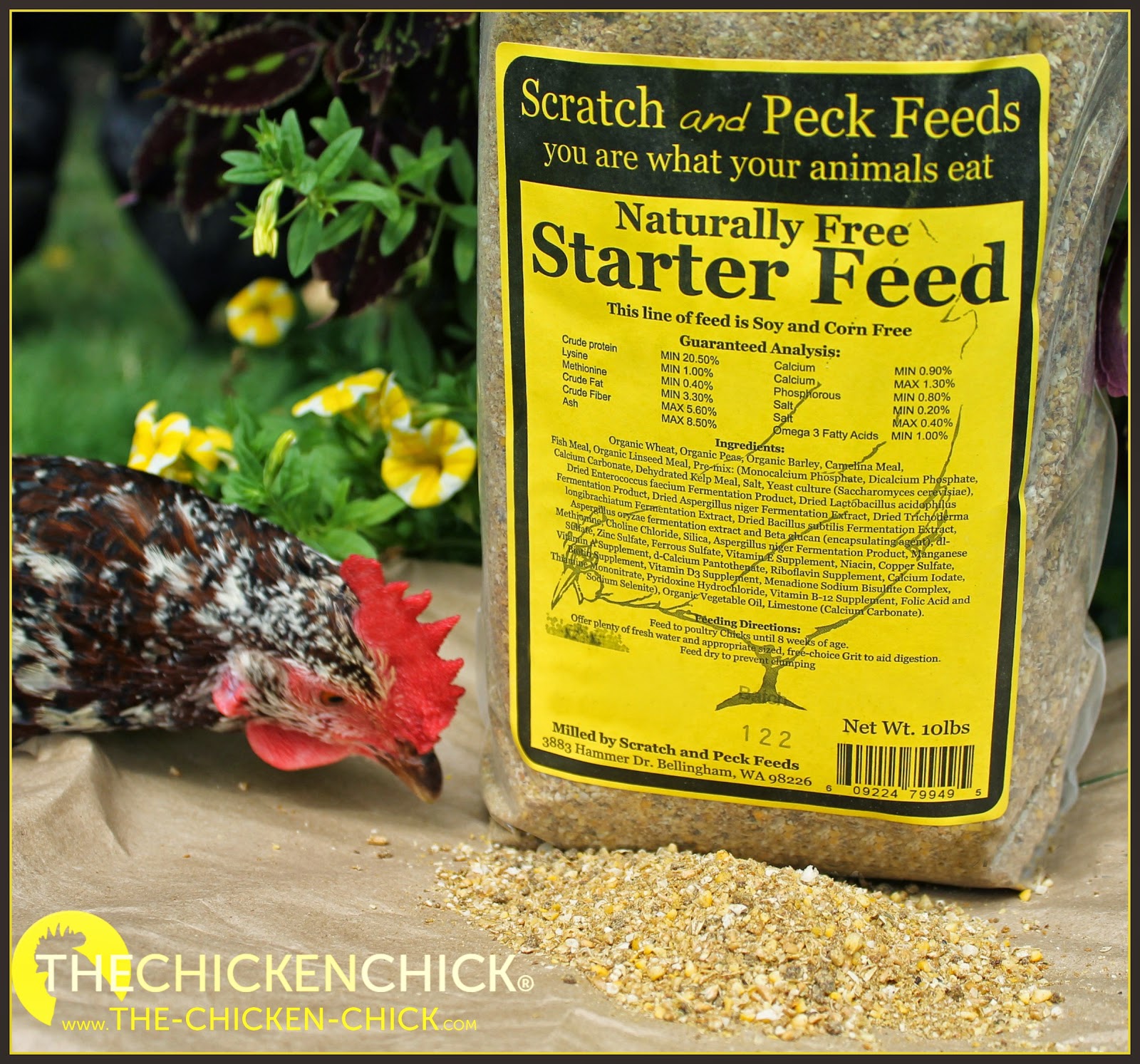This promotional image showcases a 10-pound, clear plastic bag of "Scratch and Peck Feeds" with a bright yellow and black label featuring the slogan, "You are what your animals eat." The label also highlights "Naturally Free Starter Feed," and includes detailed information about the feed's guaranteed analysis, ingredients, and nutritional value. In the lower left corner, a logo for "The Chicken Chick" is prominently displayed, along with the website "www.TheChickenChick.com." A brown and white chicken with a red comb is pecking at some of the feed scattered on a brown piece of paper laid on the ground. The scene is set against a background of green grass and various plants with white and yellow flowers, adding a natural touch to the advertisement.